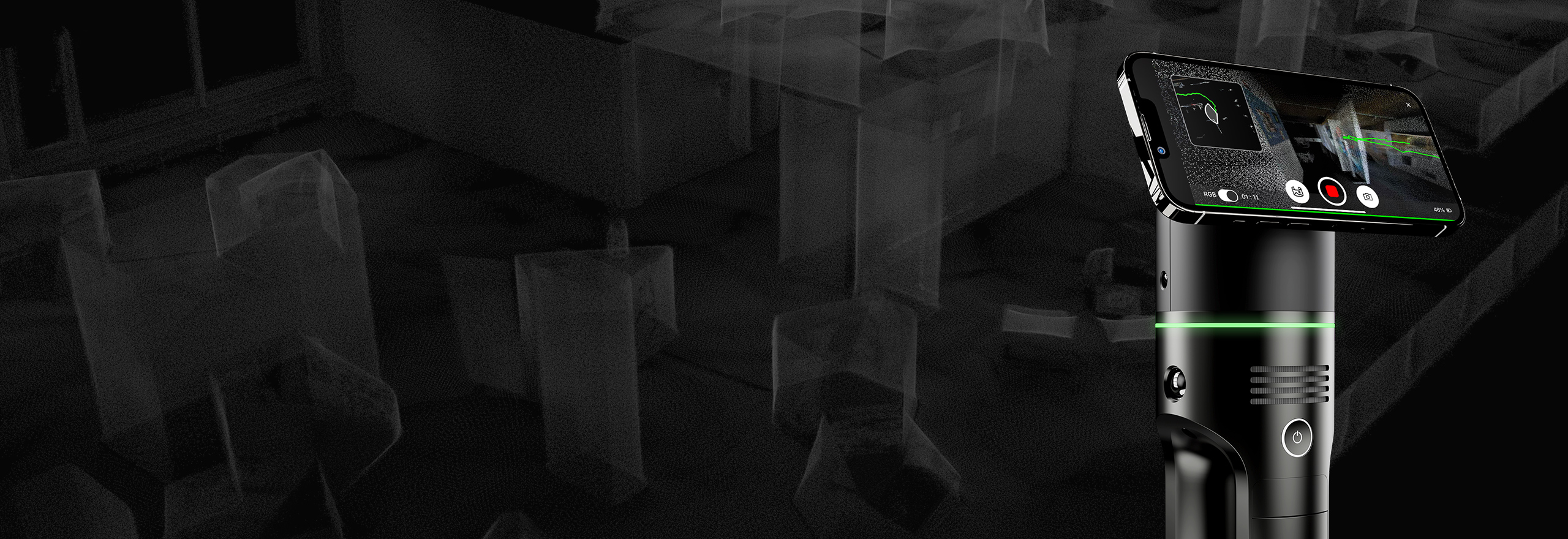The image features a predominantly dark backdrop with shades of black and gray, featuring indistinct, computerized gray shapes that resemble a 3D maze or virtual environment. On the far side of the photo, a smartphone is positioned horizontally, appearing to be recording something. It is mounted on a thick, round, and tall black stand, which has a distinctive green line running horizontally through its middle along with several buttons, including a power button at the bottom. The screen of the smartphone displays what looks like a virtual reality interface, perhaps involving green lasers darting through a hallway or maze-like space, giving a glimpse into a setting with doors, hallways, and office furniture such as desks and chairs. Interpreted as a potential recording or VR device, the setup suggests an immersive technological function, possibly for augmented reality or advanced spatial capture.